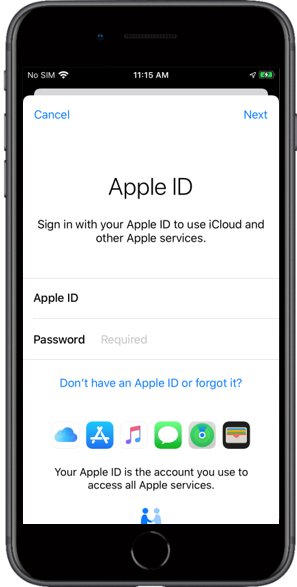The image displays a cell phone with its front screen turned on. The top section of the screen has a black background, indicating no SIM card installed with the text "No SIM" and signal bars displayed to the lower left. The current time is centered, showing 11:15 AM. On the right side, a fully charged battery icon with a lightning bolt inside indicates the phone is either fully charged or connected to a power source.

The main part of the screen is white. On the top left corner, the word "Cancel" appears in blue, while the top right corner shows the word "Next" in blue. Below these, "Apple ID" is prominently displayed in black text. Underneath this heading, a sentence reads, "Sign in with your Apple ID to use iCloud and other Apple services," also in black text. A long, straight gray line separates this from the input fields below.

The first input field is labeled "Apple ID" in black text, and it is currently empty. Below it, another input field is labeled "Password" in black text, with the placeholder text "required" in light gray to the right. Further down, in blue text, it says, "Don't have an Apple ID or forgot it?" ending with a question mark.

At the bottom of the screen, a row of application icons is displayed: a blue cloud icon, a blue square with an 'A' inside representing the App Store, a music note icon, the green messaging icon, and a black square containing white, orange, and blue colors.